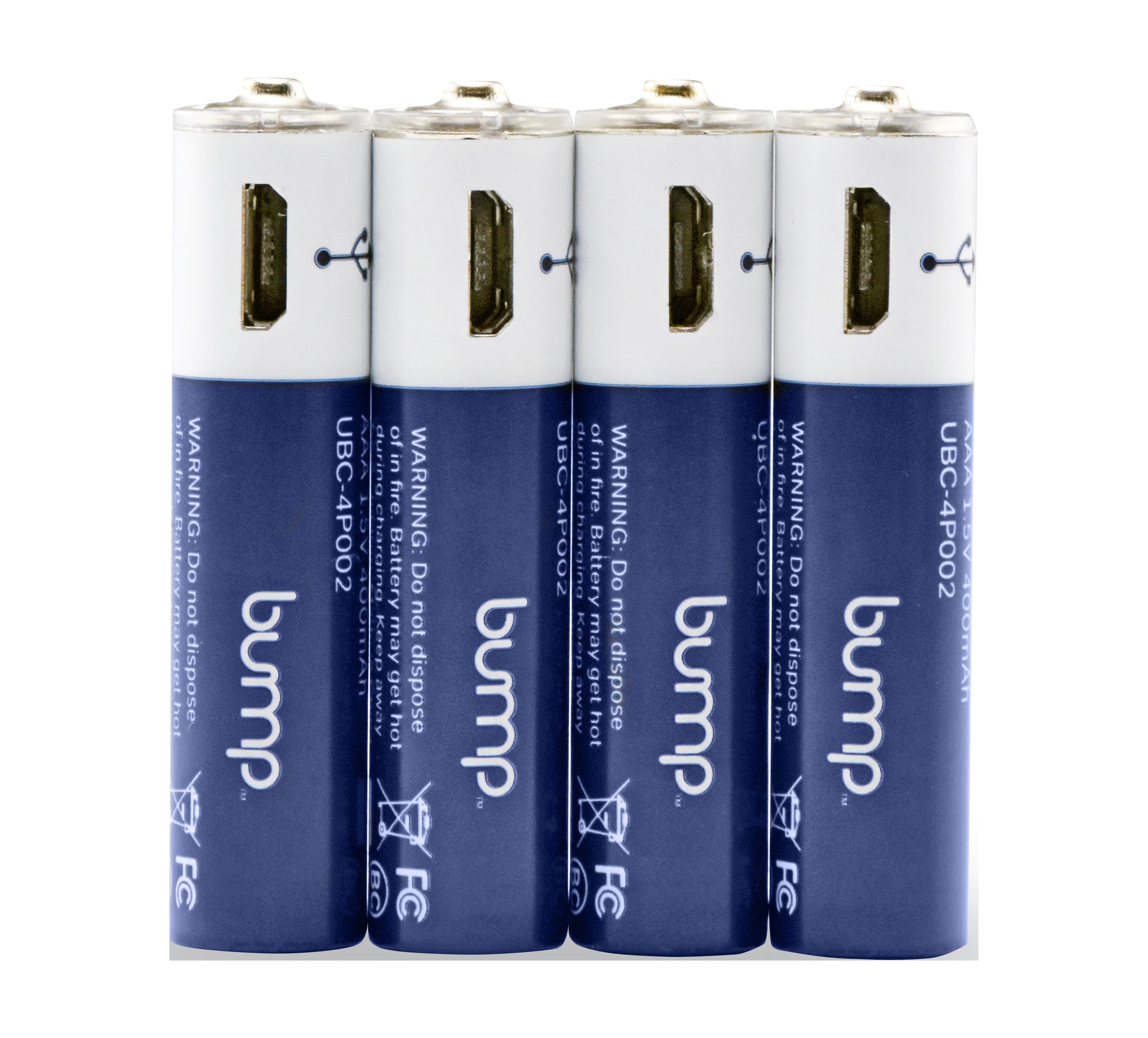The image depicts four identical rechargeable batteries branded by the company Bump, standing upright in a row. Each battery features a blue lower segment and a white upper segment with a micro USB charging port. The blue section of the batteries houses detailed white text that includes a warning: "Do not dispose of in fire. Battery may get hot during charging." Additional markings include an FCC label, a symbol indicating not to throw the batteries away, and a serial code reading UBC-4P002. The clear and white upper part of the batteries seems to have a transparent section, possibly indicating the charge level. The batteries are lined up closely together, with a distinct little knob on the end of each, giving the impression they are designed to be inserted into a device.